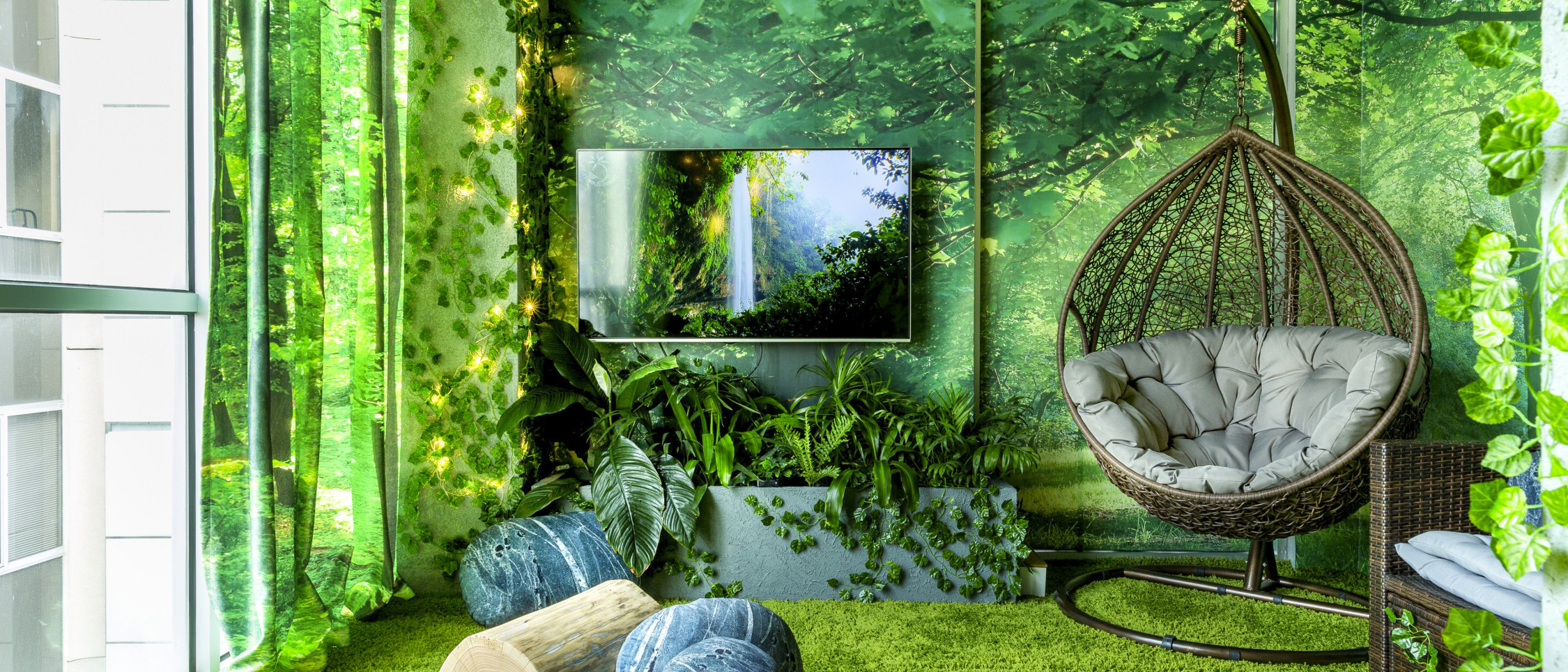This high-quality color photograph of a 1970s-inspired living room showcases a vibrant nature theme, evoking the sensation of bringing the outdoors inside. Dominating the room is an immense, photorealistic wallpaper depicting a lush forest scene, complete with a tree canopy, sunlight streaming through, and vines. The carpeting appears to be green, resembling either a lush grass or astroturf, enhancing the natural ambiance. Bright green curtains adorned with leaf patterns add to the room's verdant aesthetic.

A flat screen TV along the wall features an outdoor setting, displaying a serene video of a waterfall and green trees. Adjacent to the TV are yellow fairy lights cascading down the wall, adding a magical touch. Beneath the TV is a planter brimming with lush greenery, further reinforcing the room's botanical theme. Adding a touch of whimsy, a hanging egg-like bamboo chair, reminiscent of a 70s papasan chair, provides a cozy seating option. The floor is dotted with stone-shaped and tree-trunk-like throw pillows, inviting relaxation in this natural haven. Additional seating includes scattered cushions on the floor, creating an inviting and comfortable space.